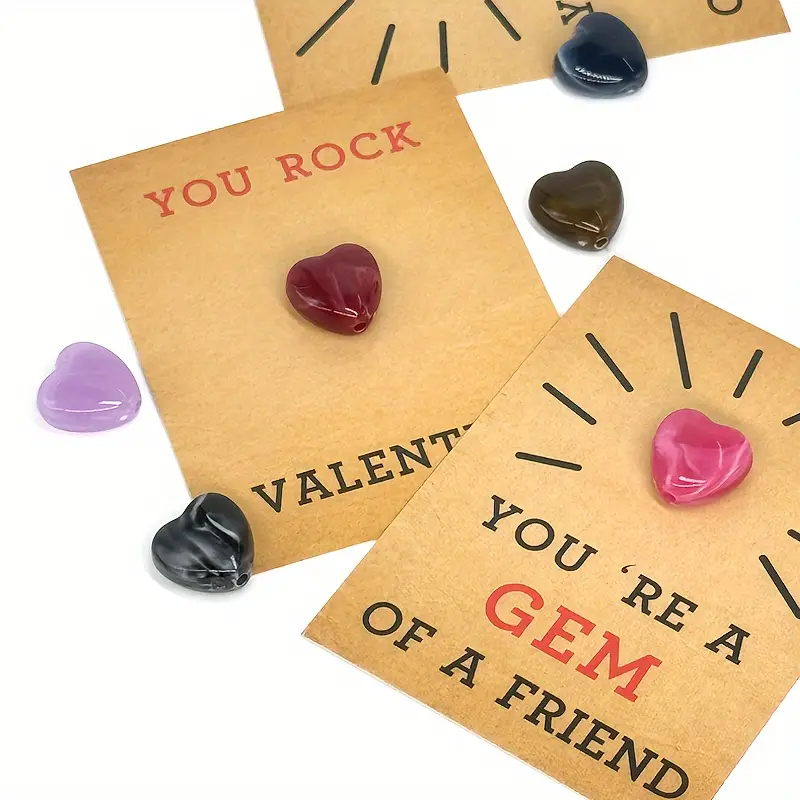This photograph features three postcard-sized, light brown cardboard Valentine's cards made from what appears to be recycled material. Each card carries heartfelt Valentine’s messages and is adorned with small, heart-shaped crystal charms in various colors. The visible cards include one that reads "You rock Valentine" with "You rock" in red letters and "Valentine" in black. Another card states, "You're a gem of a friend" with "gem" highlighted in red and the rest of the text in black. The card with "You're a gem of a friend" also features black lines radiating outwards from the pink heart crystal, giving it a sun-like appearance. Six heart-shaped crystals in total are visible: navy blue, red, purple, black with white swirls, rose, and brown. The crystals have holes drilled through them, suggesting they could be used as charms for a bracelet.